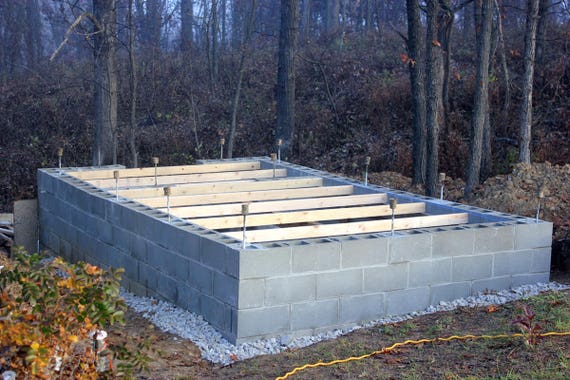The image captures the gray cinder block foundation of a rectangular building under construction in a wooded area surrounded by a border of gravel. The foundation appears complete and features rebar protruding from the top and corners of the cinder blocks. Additionally, there are seven horizontal wooden beams running from left to right across the center of the foundation. The setting includes a lightly foggy background filled with tall deciduous trees and some underbrush, with leaves scattered on the ground, indicating a possible fall season.